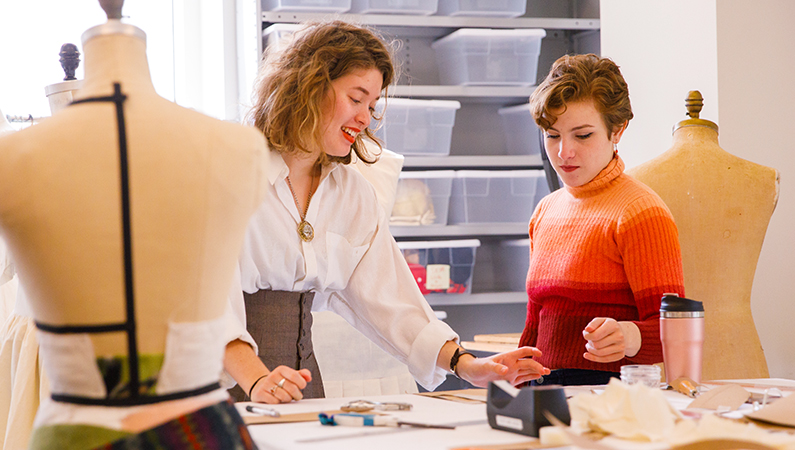Two women are engaging in what looks like a fashion design studio, surrounded by various tailoring tools and mannequins. The woman on the right has short, stylish brown hair and wears a multi-colored sweater with transitioning bands of orange and red. She’s holding out her left hand as if reaching for something on the tabletop, which is cluttered with papers, a sellotape dispenser, and pens. Next to her is a rose gold travel mug. Behind her stands an empty mannequin. The woman on the left features a white peasant blouse and high-waisted gray pants that resemble a corset under the waist. She has shoulder-length wavy brown hair and wears a necklace. She is also reaching out with her hand, seeming ready to touch something, possibly a paper on the desk. The backdrop includes grey shelves filled with clear storage bins containing various fabric swatches and accessories, and the scene includes several mannequins, some dressed partially in fabric as if mid-design, emphasizing the fashion-focused environment.